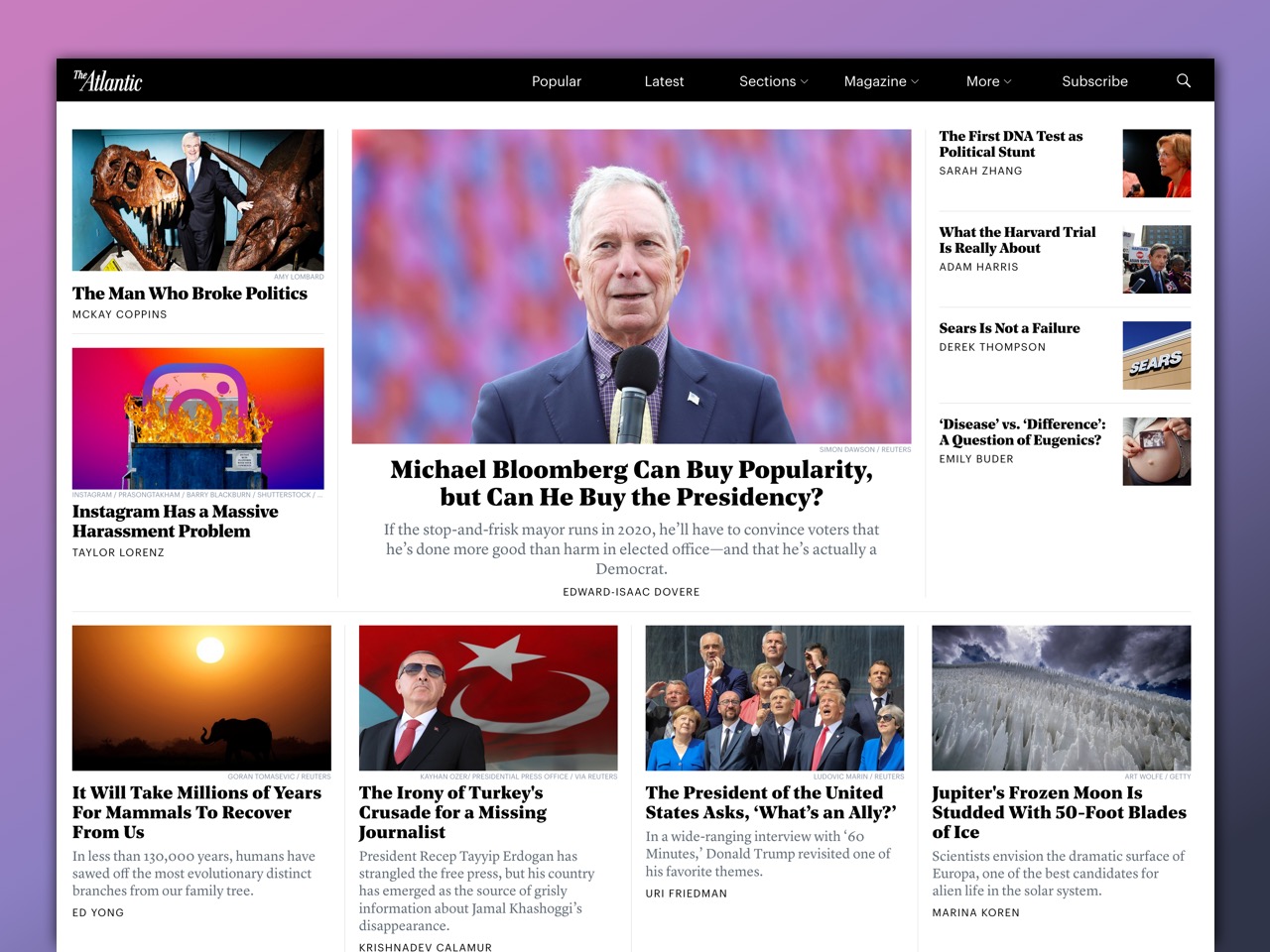This is a detailed screenshot of The Atlantic’s website. The interface features a black navigation bar at the top, with a distinctive pinkish-purple outline above it, suggesting the webpage is contained within another layer. The top menu displays links for "Popular," "Latest," "Sections," "Magazine," "More," and "Subscribe," alongside a search bar.

To the left, an image accompanies an article titled, "The Man Who Broke Politics," depicting a man standing next to what appears to be dinosaur or rhinoceros skulls. Below that, an article discussing Instagram's harassment issues is illustrated with Instagram’s icon engulfed in flames.

The central column features a headline, "Michael Bloomberg Can Buy Popularity, But Can He Buy the Presidency?" with an accompanying photo of a clean-shaven, grey-haired Caucasian man standing by a microphone, dressed in a blue shirt and jacket.

The right column highlights several headlines: "The First DNA Test as a Political Stunt," "What the Harvard Trial is Really About," "A Series is Not a Failure," and "Disease Versus Difference: A Question of Eugenics." 

The section below presents more stories: an article predicting the long-term ecological impacts of humanity, headlined by an image of the sun setting behind shadowy trees, and an article titled, "It Will Take Millions of Years for Mammals to Recover From Us." Another piece, "The Irony of Turkey’s Crusade for a Missing Journalist," is accompanied by an image of a man in front of a red flag bearing a star and crescent.

Further down, a group photograph including Donald Trump and Angela Merkel is linked to an article titled, "What is an Ally?" To the right, a picturesque shot of a grey field under a blue sky introduces an article about Jupiter’s frozen moon, "Jupiter's Frozen Moon is Studded with 50-Foot Blades of Ice." 

Each headline is paired with evocative images that complement the articles’ themes, creating a visually engaging layout.